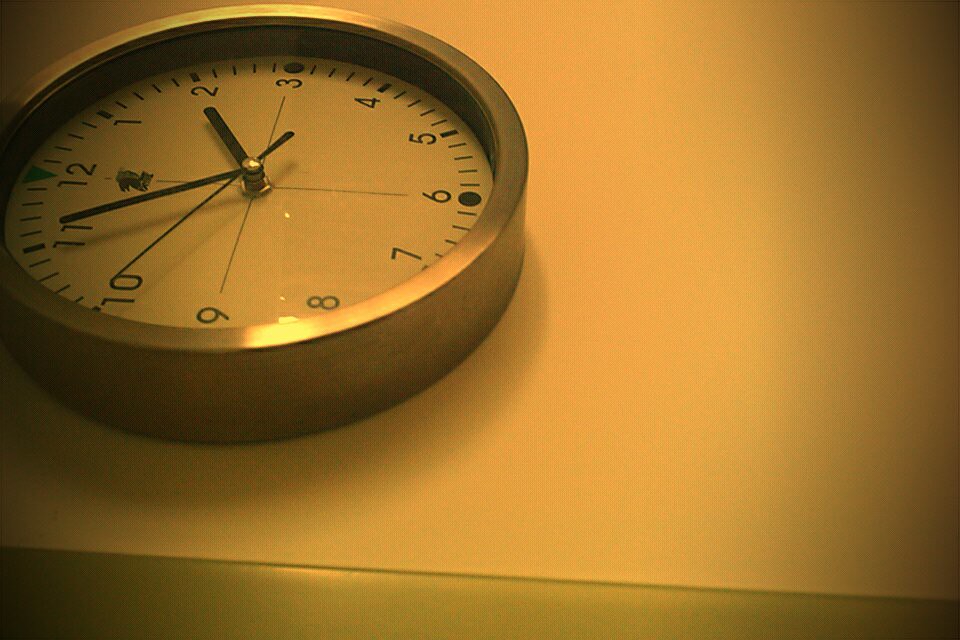This photograph captures a round wall clock with a simple, minimalist design, encased in a silver metal frame, and possibly taken at an unusual angle. The clock's face, protected by a glass cover, is white with black Arabic numerals and hands, showing the time as approximately 1:50. The image is tinted with a muted yellow-orange filter.

The clock is positioned somewhat off-center or tilted, creating a peculiar perspective where the number 9 is closest to the viewer at the bottom, and the number 3 appears at the top. This makes it seem as though the clock is turned 90 degrees to the left. There are additional black dash markers between the numerals, enhancing its simplicity.

Set against a plain white background with a subtle shadow cast towards the left, the clock image also includes a bit of olive-colored trim, possibly from a door frame, running along the left side and bottom of the frame. The shadow further suggests that the primary light source originates from the right side of the image.